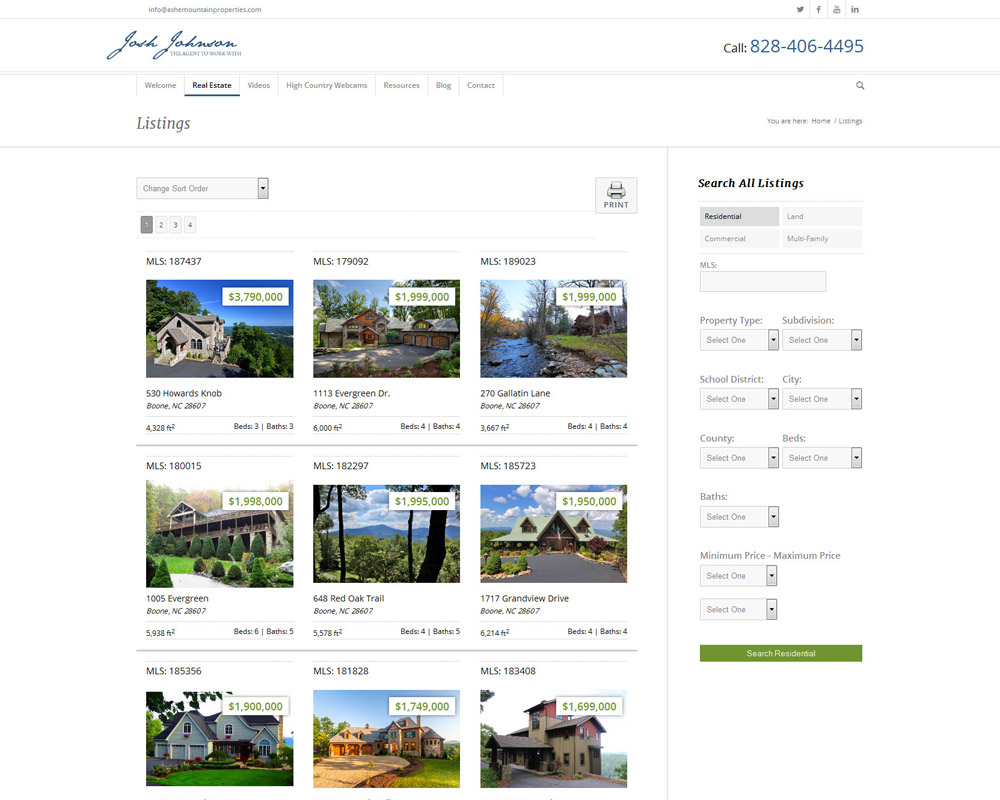The image displayed on the computer screen is a detailed page from a real estate website. At the very top left corner of the screen, there is a tiny text reading "info@AshMountainProperties.com." To the right of this email address, four social media icons are visible, representing Twitter, Facebook, an unreadable icon, and Instagram.

Below this header, there is a white background panel. On the left side of the panel, in a stylized blue script, the name "Josh Johnson" is displayed, with the subtitle "the agent to work with" written in small gray letters beneath. To the right, on the same line, the word "Call" is followed by a large, blue phone number: 828-406-4495.

Further down, a navigation bar stretches across the screen with seven menu options: Welcome, Real Estate, Videos, High Country Webcams, Resources, Blog, and Contact. These words are in gray, except for "Real Estate," which is in bold black and underlined in blue, indicating the current selection.

Under the navigation bar, in large gray script, the word "Listings" is prominently displayed. Below it, a drop-down box allows users to change the sort order of homes, paired with a button on the far right for printing the page. The site indicates that the user is on page one of four possible pages.

The main content area features a grid of nine color photographs of homes, organized in three columns and three rows. Each listing includes the MLS number, price, address, square footage, number of bedrooms, and number of bathrooms. The homes showcased are luxurious, with prices well over a million dollars, the highest being close to four million dollars.

To the right of the home listings, there is a vertical panel that lets users refine their search criteria. This panel includes options for selecting property type (Residential, Land, Commercial, and Multifamily), school district, county, subdivision, city, number of bedrooms and bathrooms, and minimum and maximum price. At the bottom of this panel is a green "Search Residential" button designed to filter the real estate listings based on the entered search attributes.